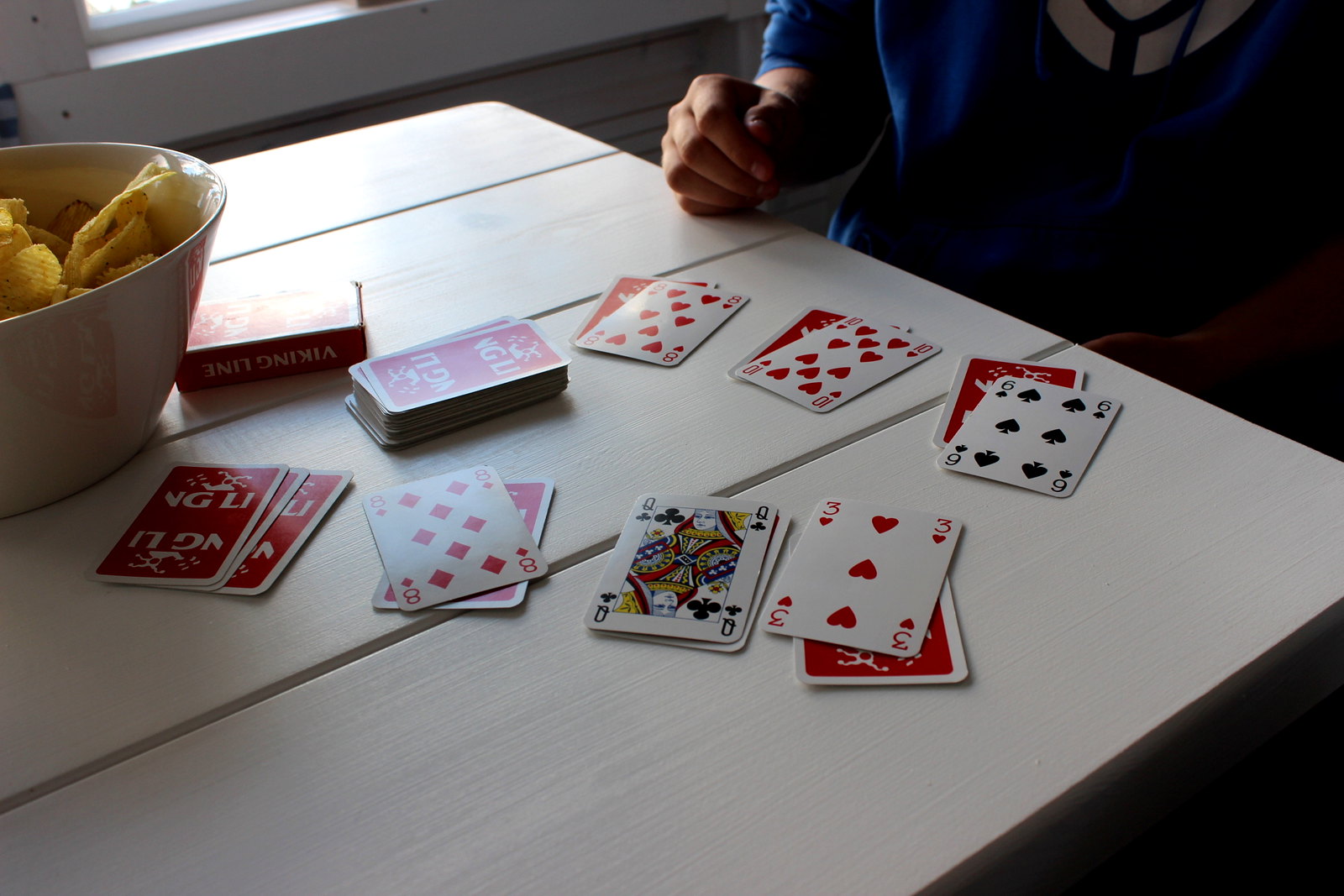In a quaint cottage-style kitchen, a wooden table painted white serves as the stage for a serene game of cards. Opposite the viewer, a young adolescent, casually dressed in a dark blue hoodie adorned with a white logo and two dangling drawstrings, is deeply engaged in arranging cards. The cards, emblazoned with the 'Viking Line' logo, are meticulously set in two rows on the table, and the box they came in is placed on the right-hand side. The scene suggests a game of solitaire, though the specific game remains a mystery. The adolescent's right hand rests on the table, while the left hand lies on their lap, hinting at a relaxed state. In front of them, a beige ceramic mixing bowl brimming with crinkle-cut potato crisps adds a touch of indulgence to the moment. Sunlight filters softly through the kitchen window, casting a warm glow over the idyllic setting. This tranquil scene captures a moment of peaceful relaxation and simple enjoyment.